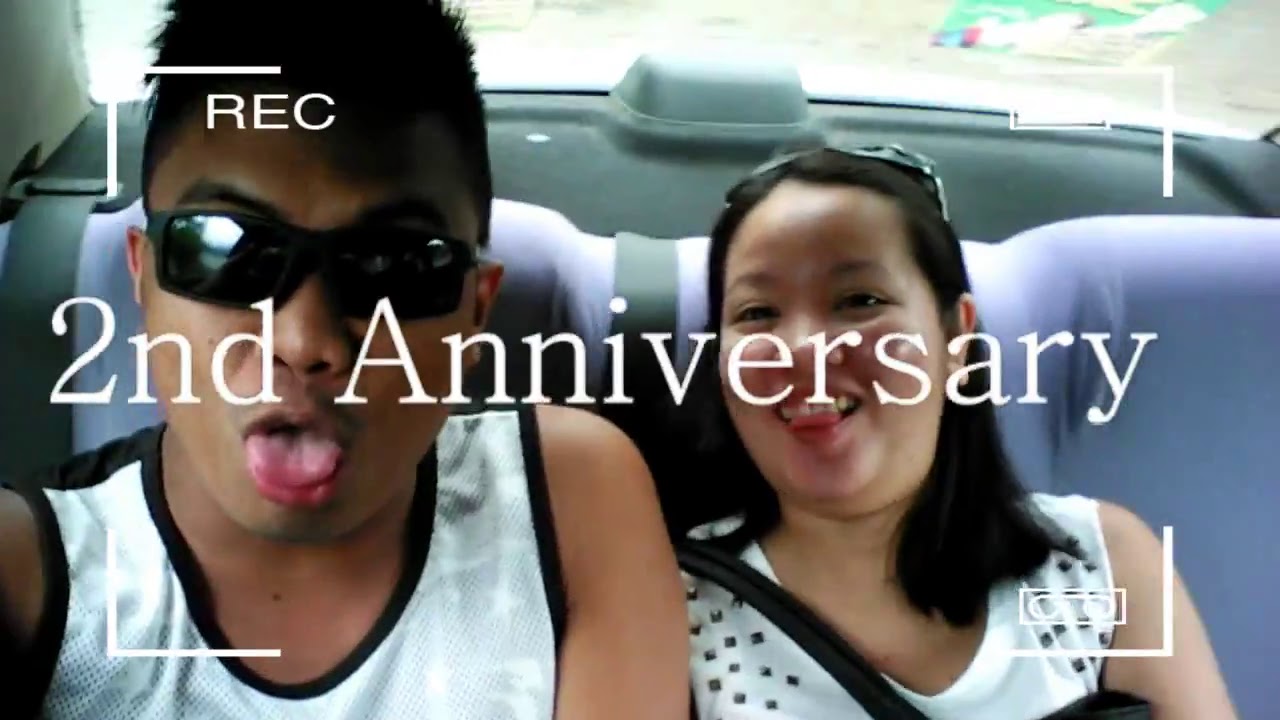This color photograph captures a joyful moment of a couple celebrating their second anniversary. They are seated side by side in the backseat of a car with blue upholstery and a visible gray shelf through the rear window. The image is overlaid with a white camcorder-style frame, featuring the text "REC" in the upper left corner and "second anniversary" prominently across the middle. 

On the left is a brown-skinned man with dark sunglasses obscuring his eyes, black hair, and a white tank top with black piping around the neck and arms. He playfully sticks out his tongue, leaning slightly forward toward the camera. Beside him, on the right, is a brown-skinned woman with shoulder-length black hair. Her sunglasses rest atop her head, and she, too, sticks out her tongue with a smile. She wears a white tank top adorned with black dots and what appears to be diamond-shaped beading on the sleeves, along with the visible strap of a handbag slung over her shoulder. Both share a carefree and celebratory demeanor, perfectly captured in this vibrant and intimate snapshot.